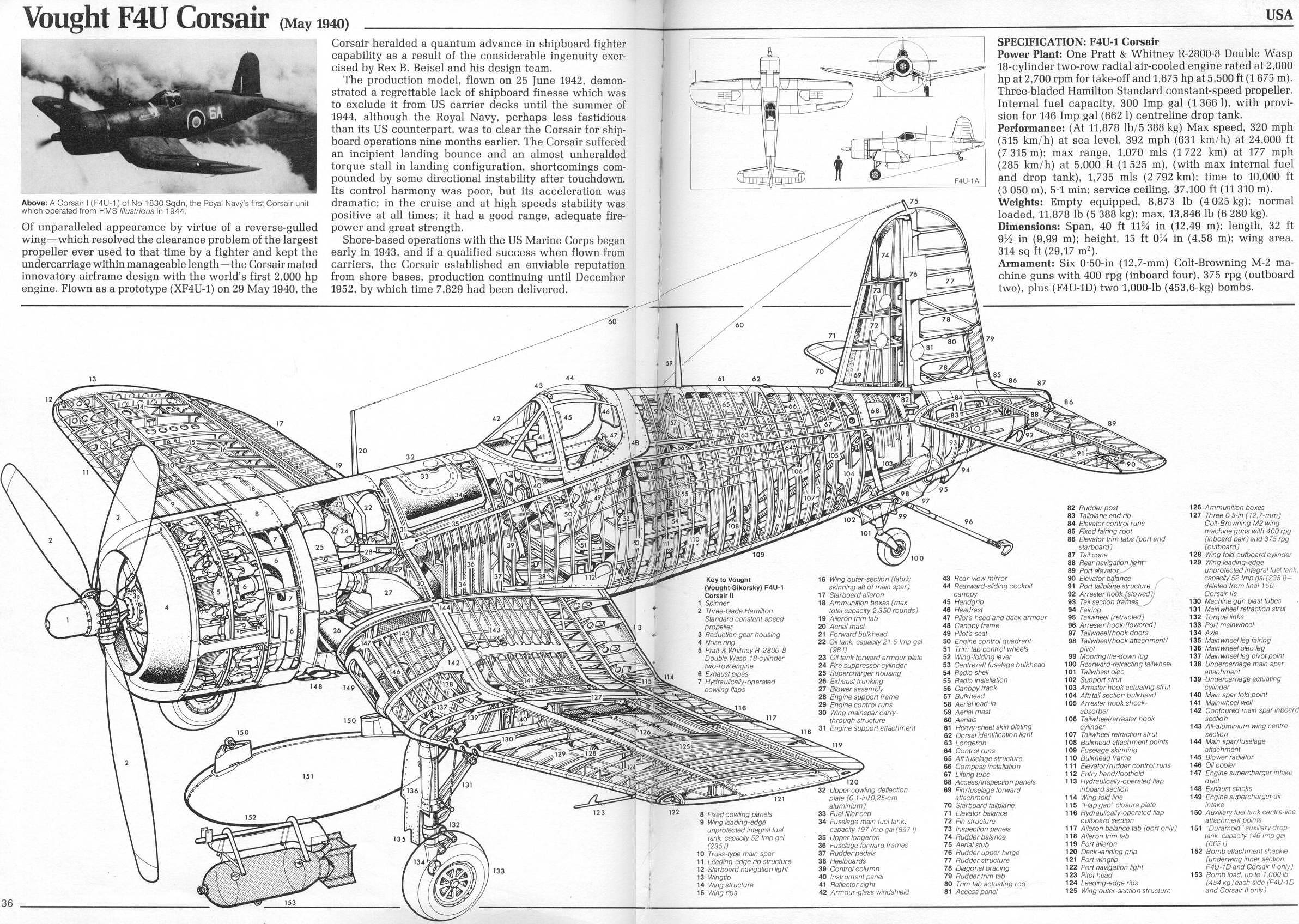The image depicts a pair of interior pages from a book or magazine featuring an extensive article and detailed schematic of the Vought F4U Corsair, a World War II fighter plane, dated May 1940. The top portion of these pages contains an in-depth article complete with specifications such as the Pratt & Whitney power plant, performance metrics, weight, dimensions, and armament details including bombs. It is comprehensive and filled with technical data, suggesting a highly informative piece.

The bulk of the pages is dominated by an incredibly detailed black-and-white cutaway illustration of the Corsair, showcasing the internal structure down to the individual struts, pieces, engine parts, flaps, and wires. The propeller faces to the left, and the tail points slightly upward to the right. The drawing exposes the plane's skeleton, revealing intricate details like ridges, the engine location, and a bomb or gas tank positioned between the wheels. Notably, the plane's tail dragger style and aircraft carrier hook are visible, emphasizing its naval use. 

Around this detailed illustration, numbers label approximately 150 different parts, providing a highly technical guide to the plane's components. Accompanying these labels are detailed explanations listed to the right of the drawing. A smaller, actual photograph of the Vought F4U Corsair is positioned in the top left corner, offering a visual reference of the plane's exterior. This meticulous combination of visual and textual information paints a comprehensive picture of the Vought F4U Corsair.